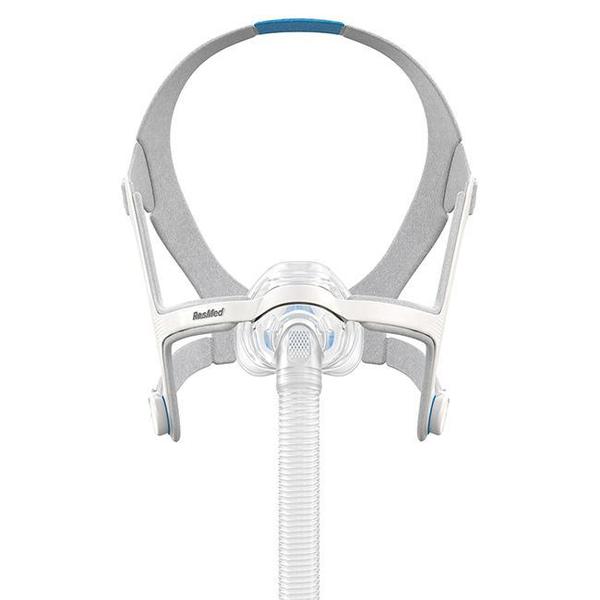The image shows a detailed view of an oxygen or gas mask apparatus, likely a CPAP machine, designed for breathing assistance during sleep. The device features a roughly triangular clear plastic cup that covers the nose and mouth, with a ribbed plastic tube extending from it for airflow. The mask is secured by a framework made from a combination of plastic and metal, along with soft straps to fit around the head comfortably. The front bar of the framework, which has a faint, small logo that appears to be "ResMed" or a similar brand, runs across the front of the face. The setup includes a gray band and a white strip that further secures the mask, all set against a predominantly white background with some blue tinting. The intricate design includes loops and clips to ensure a snug fit around the head and neck.